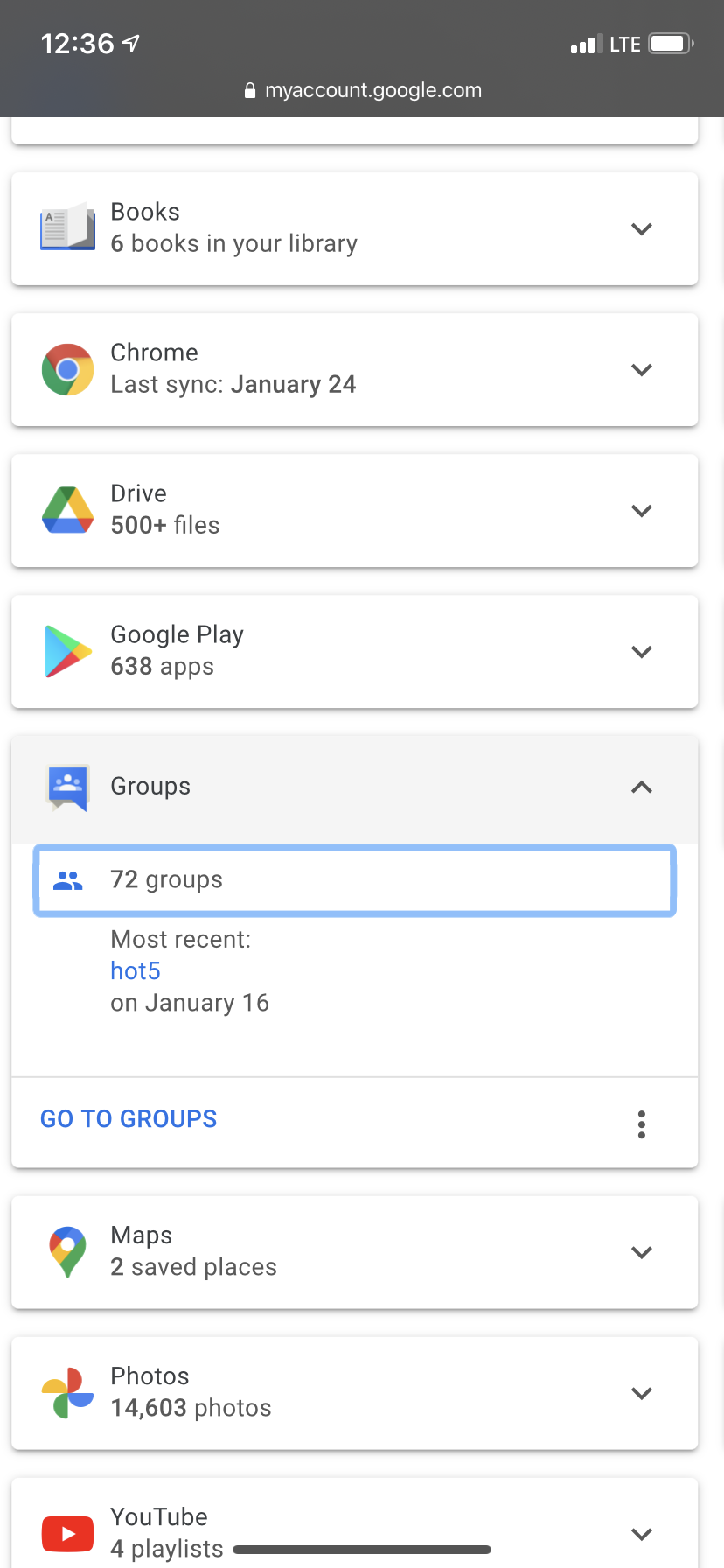The image features a white background with a gray header at the top. Within the gray rectangle at the top, the URL "1236 myaccount.google.com" is displayed. Below the header, there are several smaller rectangles:

1. The first rectangle highlights the "Books" section, showing "6 books in your library." It includes a down arrow for further options.
2. The next section is "Chrome," with the text "Last sync January 24th" in bold.
3. For "Drive," it displays "500+ files" accompanied by a down arrow.
4. The "Google Play" section mentions "638 apps," also with a down arrow.
5. The "Groups" section is enclosed in a gray bar, stating "72 groups," with the note "Most recent: 'Hot Five', on January 16th" in blue text. This area includes an up arrow and a "Go to groups" link in blue, followed by three vertical dots.
6. In the "Maps" section, it notes "2 saved places" along with a down arrow.
7. The "Photos" section shows "14,603 photos" with a down arrow.
8. Finally, the "YouTube" section mentions "4 playlists" and includes a down arrow.

At the bottom of the layout, there is an additional gray bar situated in the middle.